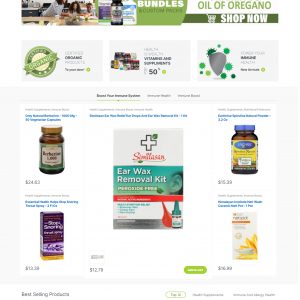Screenshot from a Healthcare Remedies Website: This image, captured from a website specializing in herbal healthcare solutions, showcases a variety of natural remedy products. Centrally featured is an earwax removal kit, prominently advertised as utilizing 100% natural ingredients. Adjacent to this, the website offers oil of oregano with a convenient 'Shop Now' option. Also available are various capsules derived from natural omega oils. A notable highlight across the site is the repeated assurance of products being 100% organic, emphasized in green font. Unfortunately, specific pricing details for these items are indiscernible due to the image's heavy pixelation.